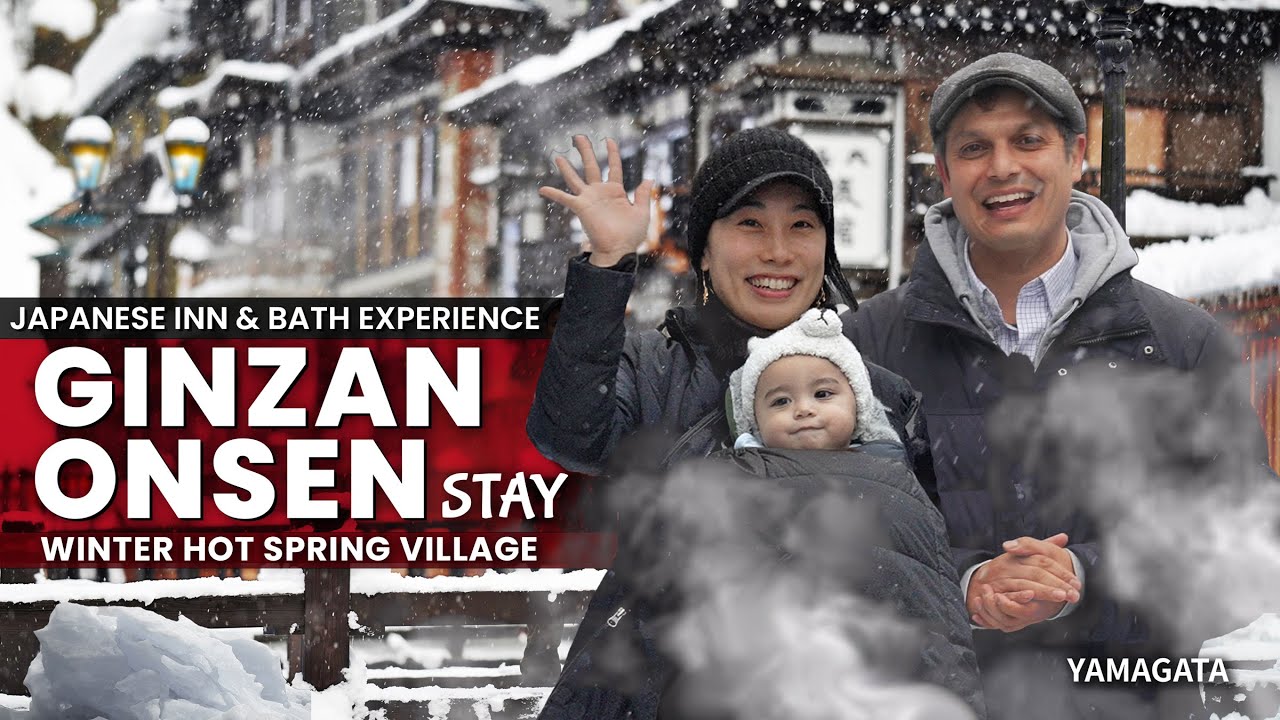The image is a real photograph, reminiscent of something you'd find in a magazine, serving as a YouTube video thumbnail. It promotes a Japanese inn and bath experience titled "Ginsen Onsen Stay, Winter Hot Spring Village." On the right side of the image, there's an American gentleman in his late 40s wearing winter gear. To his right, an Asian woman, presumably his spouse, also dressed in winter attire, holds their child, who is donning an adorable white bear-shaped hat. Both adults are smiling and waving at the camera, encapsulating a warm, welcoming vibe despite the cold setting. Snow falls both in the background and foreground, contributing to the wintery ambiance. The background also features the inn itself, a predominantly black structure accented with white. The text "Yamagata" appears at the bottom right of the image, likely indicating the video's location.